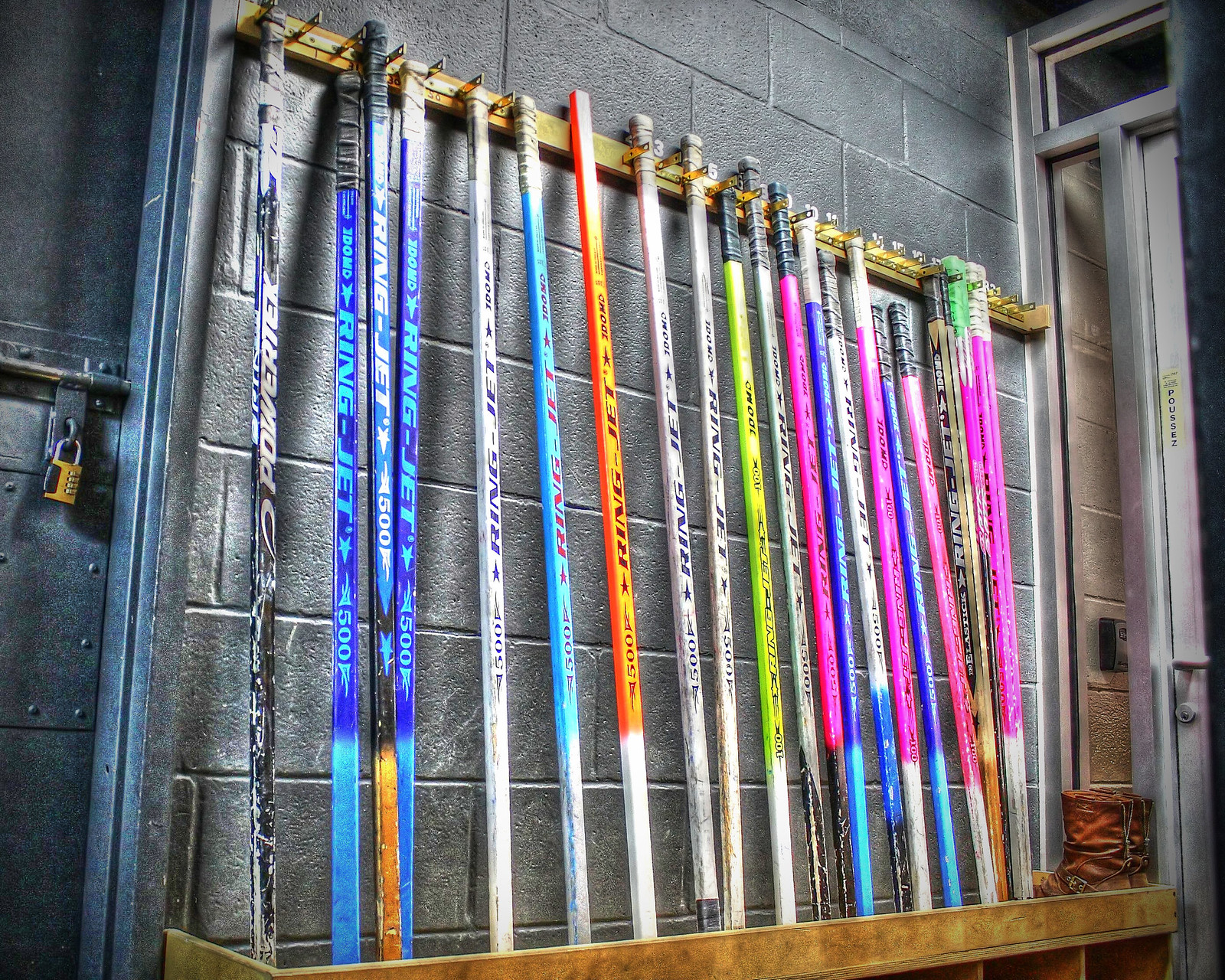This indoor image captures a gray, spray-painted brick wall against which a collection of colorful hockey sticks are arranged. These hockey sticks, varying in hues such as black, blue, white, orange, yellow, neon green, bright pink, and very dark blue, are seen leaning against the wall, secured by a wooden beam at the top and possibly at the bottom, although the lower part is not visible. Some sticks display brand names like "Power Tech" and "Ring Jet 500." On the left side of the image, there is a door with a gold padlock attached, and on the right-hand side, part of a clear glass door with a white handle is visible. In the lower right-hand corner, a red object can be seen, though its exact nature is unclear.